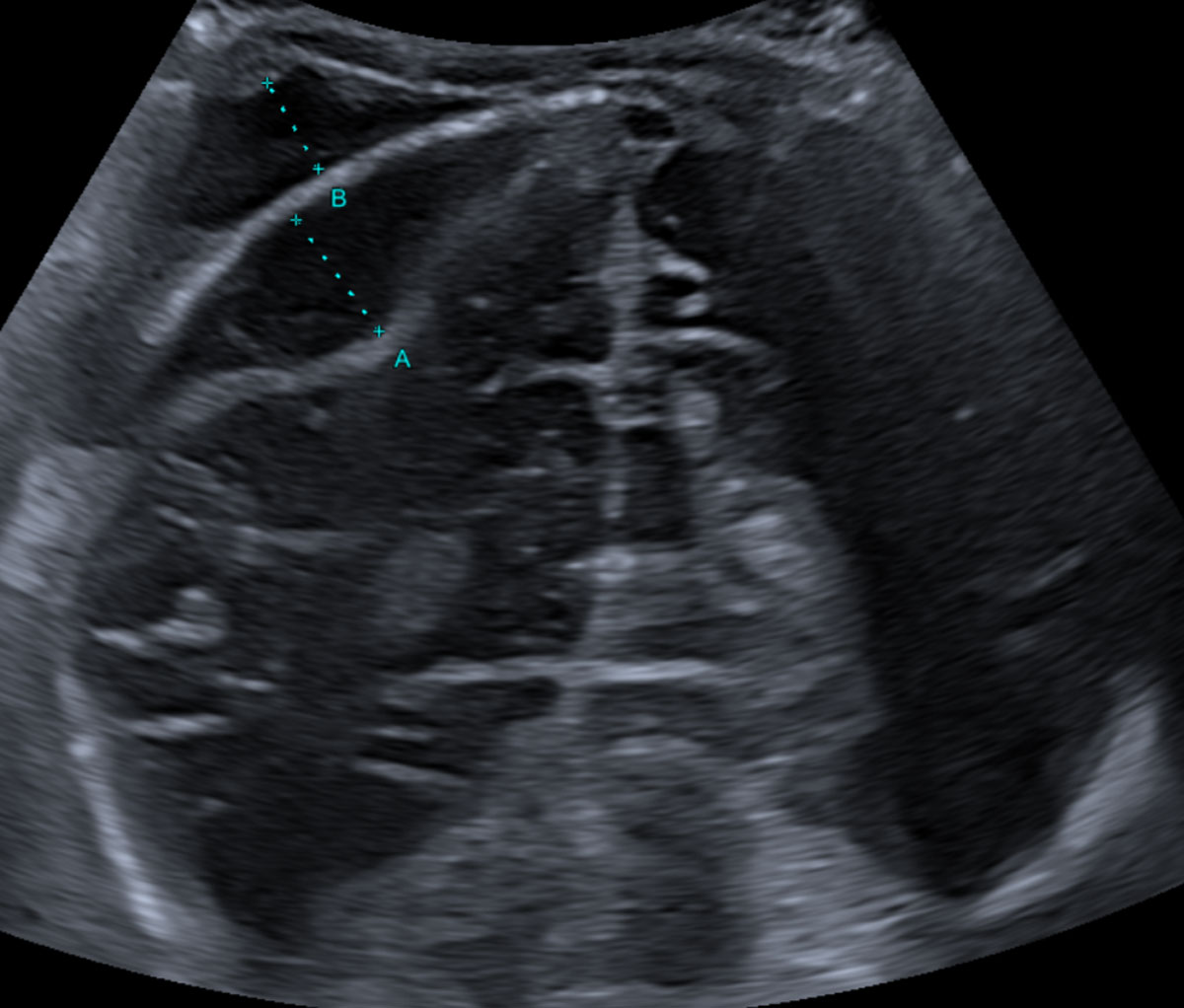The image is a grayscale ultrasound featuring a real-time black-and-white sonographic scan. In the upper left corner, there are two labels, "A" and "B," each marked with a series of dots leading to a specific point denoted by plus signs. These labels highlight different structures, potentially bone or tissue, although the exact details are unclear due to the grainy quality of the image. The central section of the ultrasound shows more bodily structures extending downward, but their precise nature is indistinct. The background of the scan is a solid black gradient, emphasizing the highlighted points marked by "A" and "B." Overall, the image is a scientific ultrasound depicting parts of a human body, though it is not distinctly clear which specific features or organs are being shown.